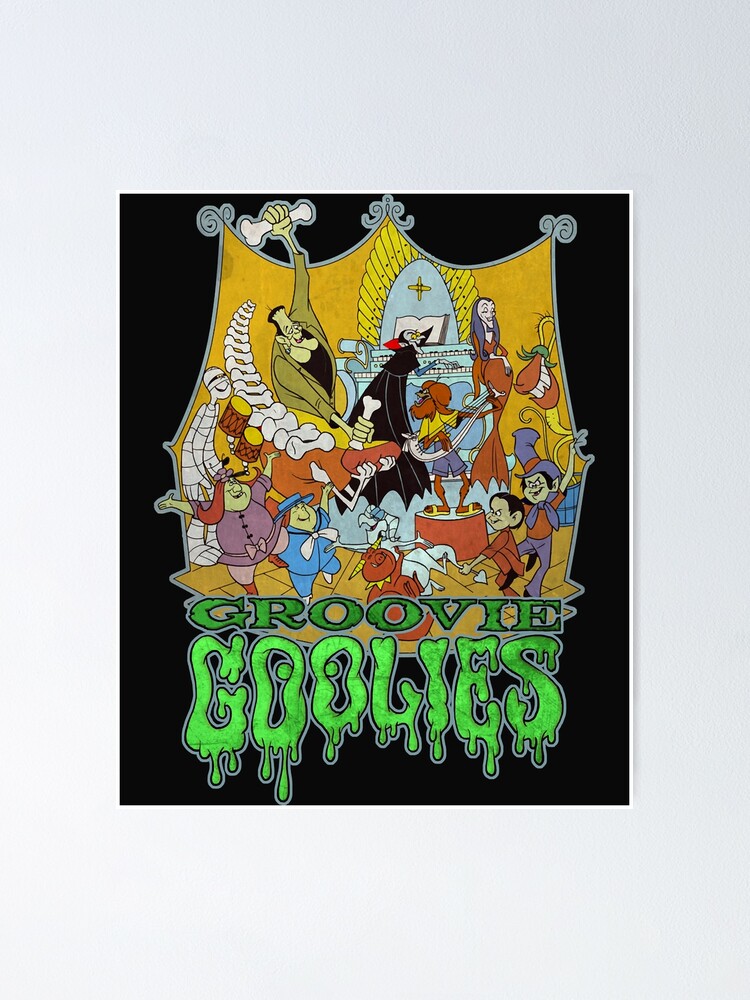This vibrant poster set against a black background with a thin white border depicts a lively Halloween party scene. In the foreground, various children are energetically dancing in costumes. Center stage, a Dracula-like character is engrossed in playing a light blue piano, accompanied by a Morticia Addams look-alike standing beside him, cradling her belly. The top left corner features a Frankenstein-inspired figure holding a bone in each hand, seemingly playing a bone xylophone. To his far left, a mummy wrapped in white bandages passionately plays yellow drums. The entire scene is brought to life with a yellowish-gold backdrop that contrasts the grayish white border surrounding the illustration. At the bottom, the playful green text "Groovy Ghoulies" splashes across the poster, with the word "ghoulies" mimicking a dripping paint effect reminiscent of the Goonies logo. This detailed tableau captures the essence of a quirky, animated band of ghoul characters, each contributing to the festive atmosphere with their musical talents.